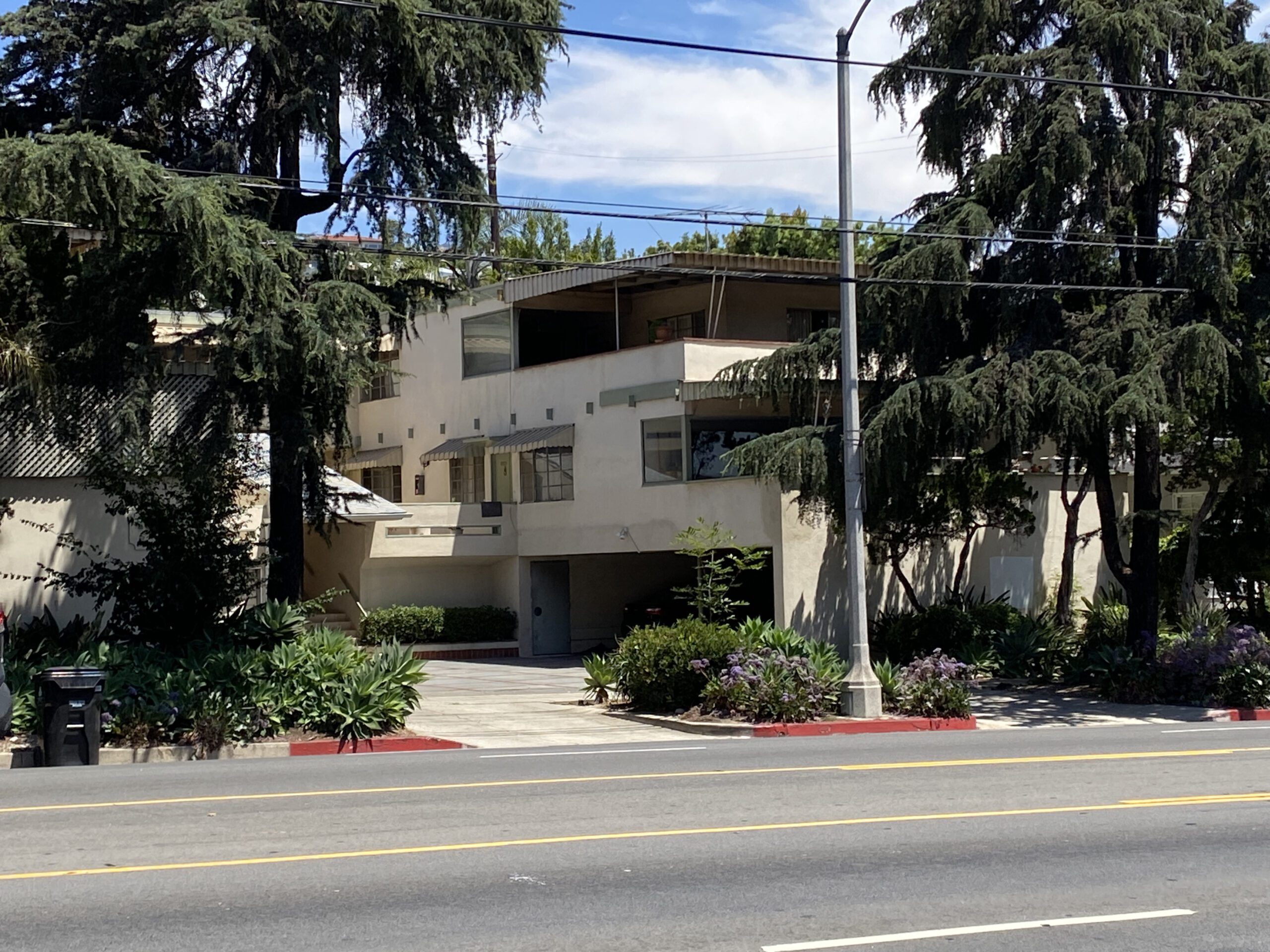This outdoor photograph captures a city street scene from the perspective of someone standing across the street, looking at a condo complex. The bottom of the image features a road with yellow and white street lines and a median adorned with flowers and bushes, including some purple blossoms. A streetlight protrudes from this median, illuminating the area. Tall, dark green trees flank a driveway and sidewalk with additional plant life. The condo complex in the background is around three stories high, with multiple windows on each level, a garage, and a door at the ground level. There's also a staircase on the left, leading to the entrances of several units. 

The cream-colored building exhibits a boxy, geometric design, possibly made of stucco, and appears very modern. Another similar structure is partially visible on the left, obscured by trees. Overhead, telephone and electrical wires crisscross the clear, blue sky, marked by a few white clouds. The scene is rich with greenery, with nearly half the photo dominated by various trees and plants, highlighting the condo's urban yet lush setting.